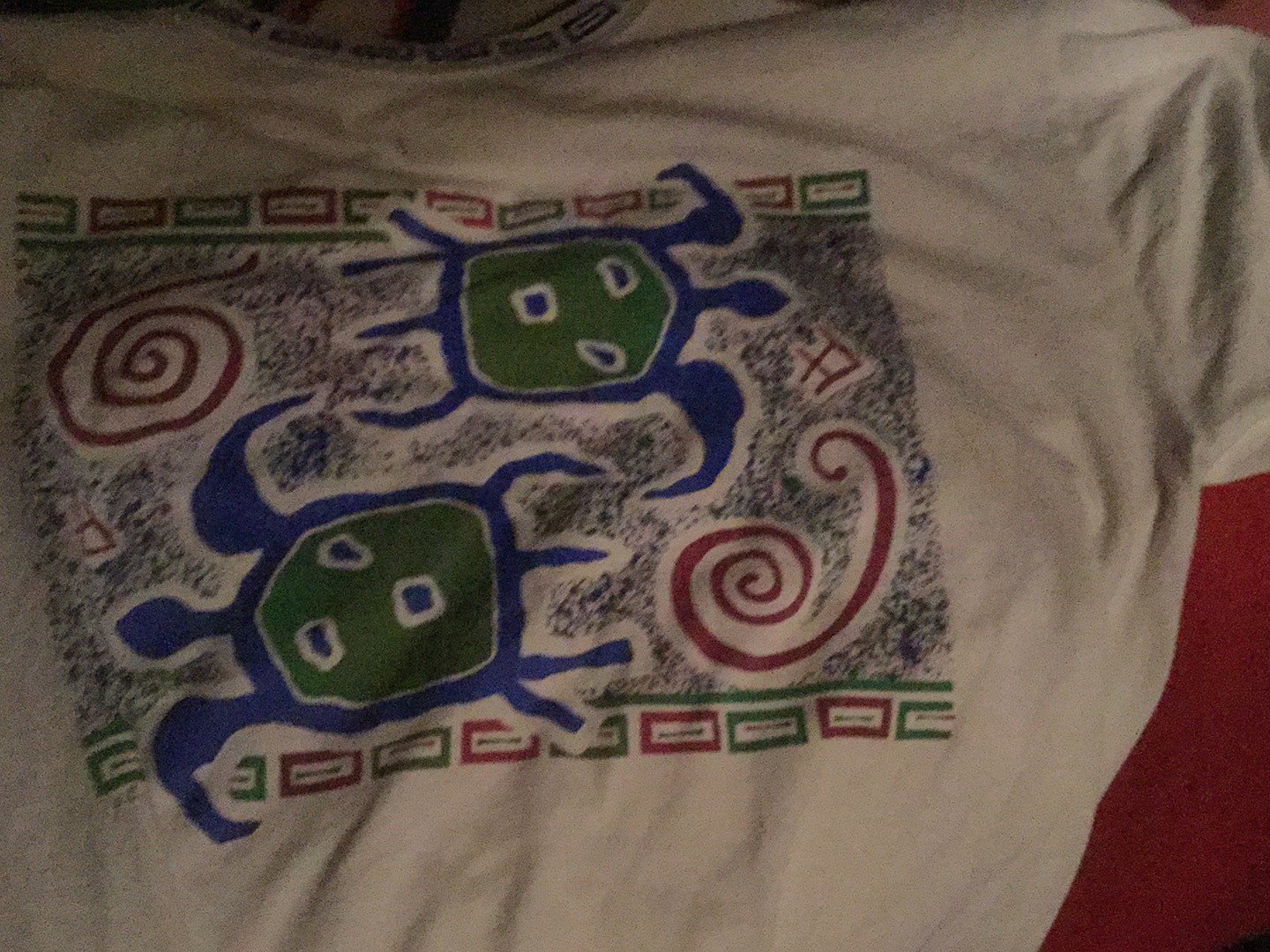This image depicts a slightly wider-than-tall photograph of a t-shirt, laid flat on a surface that reveals a hint of red at the lower right corner, suggesting the underlying backdrop. The t-shirt is either white or light-colored and prominently features an intricate graphic on its front. The artwork appears to draw inspiration from Australian or tribal designs, showcasing two crab-like figures with blue bodies, green faces, and square-shaped mouths. These crabs have four legs each and possess either elongated ears or claws, with a small protuberance atop their heads. Positioned horizontally and facing opposite directions, the figure at the top faces right, while the one at the bottom faces left. The design includes two red spirals and various additional background elements that contribute to its detailed appearance. Along the collar, a series of black rectangles form a pattern that frames the top of the shirt, adding a unique touch to the overall design.